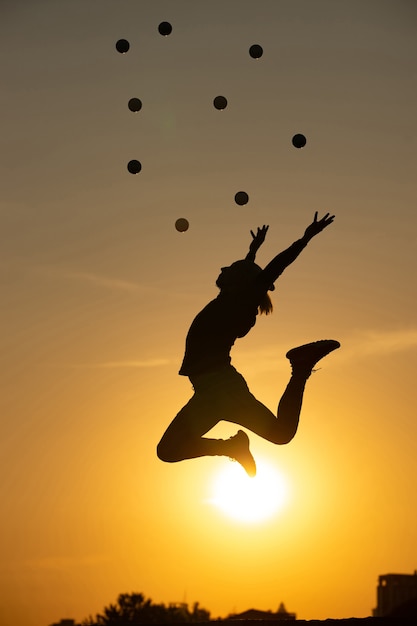In this color photograph taken outdoors, a silhouetted young woman is captured leaping into the air against a yellow sky. She is facing left, with her arms stretched above and behind her head, and her legs bent at the knees, kicked up behind her. The sun sits low in the sky, glowing brightly with a hazy aura caused by thin, high-altitude clouds. Surrounding her, nine small balls are being thrown into the air, suggesting she released them during her jump. Visible at the bottom of the image are the dark silhouettes of treetops and a few distant buildings, adding depth to the scene. The woman is wearing sneakers, leggings, and a shirt, though their colors are indistinguishable in the silhouette.